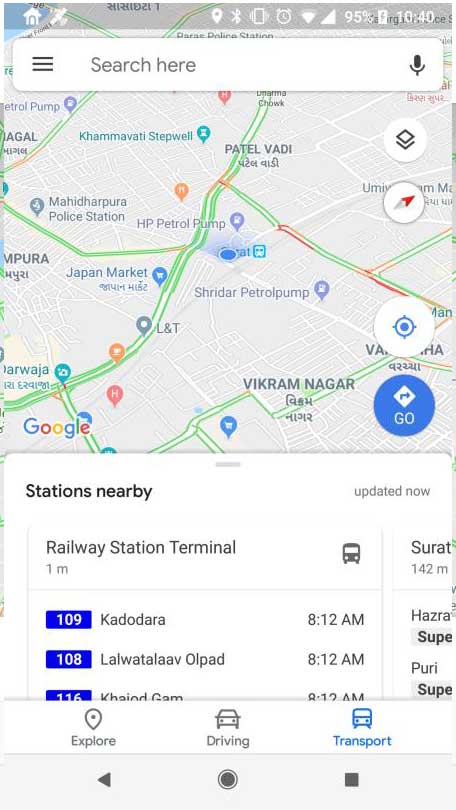**Detailed Image Description:**

At the top of the image, there is a gray top bar. On the top left corner of this bar, a white outline of a house icon is visible. To the far right side of the bar, the time reads "10:40". Next to the time, there is a battery icon showing 95% power. Beside the battery icon, the Wi-Fi signal is nearly full. Additionally, a clock icon is located near these elements.

Just below the gray top bar, there is a white search box with a few elements inside it. On the left, there are three black horizontal lines. In the center, it reads "Search here" in black font. On the right, there is a black microphone icon.

Beneath the search box, a map with a gray background indicating housing areas and green lines representing roads is shown. On the right side of the map, a white circle with a triangle and line underneath it is visible. Below this, a secondary circle features red and gray triangles pointing in opposite directions. Another nearby circle contains a search button with a blue center and a blue outlined circle. The last circle beneath displays a blue background with "Go" written in white font alongside a white triangle-arrow pointing to the right.

Overlaying the map to the left, the traditional Google logo is presented, with the "G" in blue, the first "O" in red, the second "O" in yellow, another "G" in blue, an "L" in green, and "E" in red.

Beneath this logo, a white background box with black font text states "Stations Nearby" on the left. Below this header, it reads "Railway Station Terminal" and "1 minute". To the right, the text "Updated now" is present along with an image of a grayish bus. 

Separated by a line, the text "SURAT" appears, followed by "142M". Below this are three blue boxes containing bus route details:
1. "109 Kadaria, 8:12 AM" in black font.
2. "108 LALWATALAAVOLPAD, 8:12 AM".
3. "116" which is slightly cut off.

At the screen's bottom, three options read from left to right: "Explore", "Driving", and "Transport". These are accompanied by their respective icons - an exploration icon for "Explore", a car image for "Driving", and a blue bus icon for "Transport".

Finally, the bottom gray bar displays a black arrow pointing to the left, a black circle in the middle, and a black square on the right.